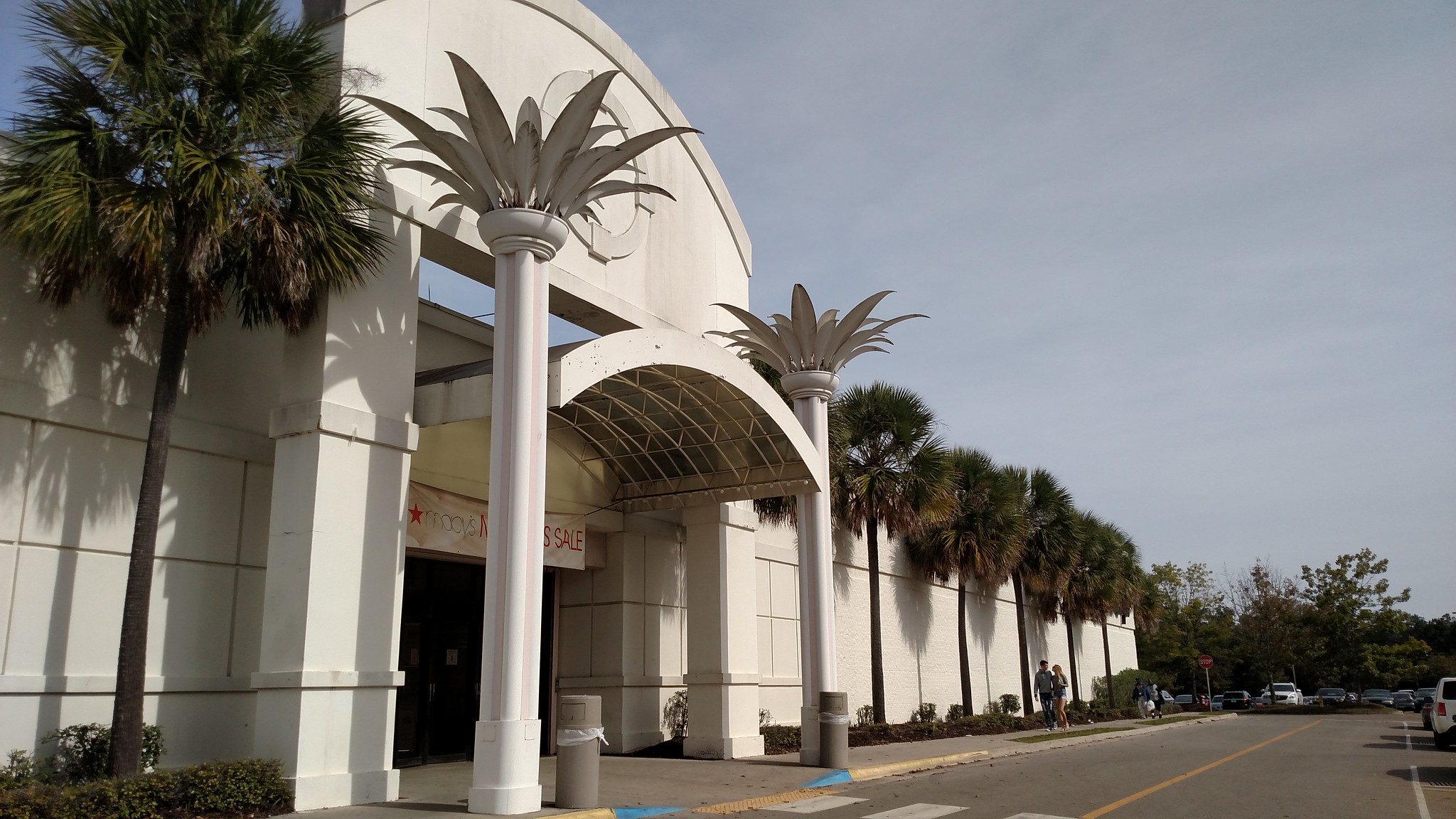The image depicts the entrance of a large, modern building, which appears to be a shopping mall. The prominent feature is a large banner advertising a Macy's sale, suggesting that Macy's is one of the anchor stores within the mall, although there is no direct signage confirming this. The entrance is flanked by six tall palm trees, which line the facade of the expansive structure. A road runs parallel to the building, and a car is visible in the distance. The scene is bathed in natural daylight under a very clear sky, signifying that the photo was taken on a bright, sunny day.